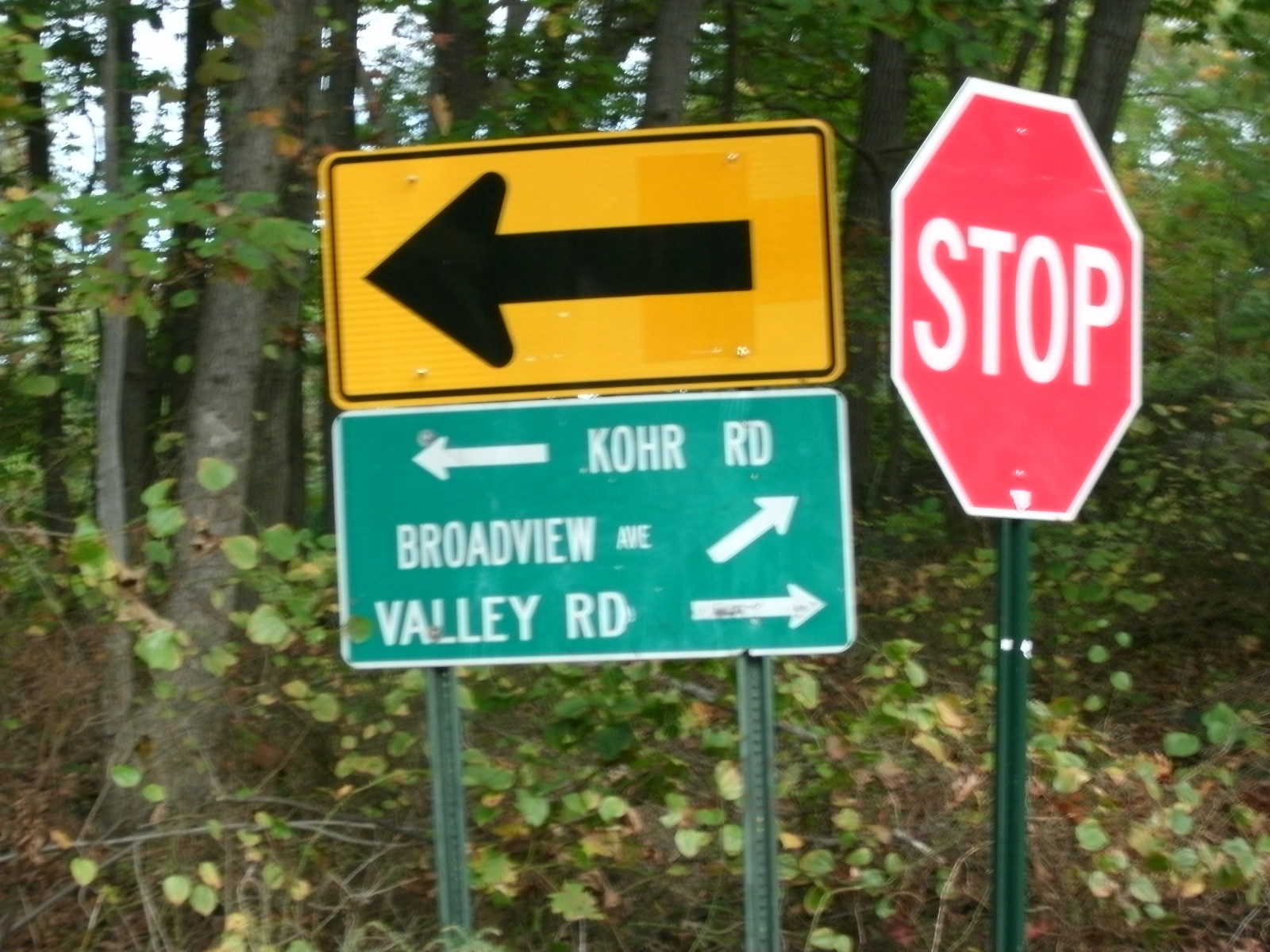In the center of the image, a cluster of street signs stands against a backdrop of a dense forest with tall, slender trees adorned with green leaves and patches of brown foliage. Dominating the scene is a yellow sign with a black arrow directing left. Just beneath it, attached to the same set of metal poles, is a green sign with white text indicating "Coor Road" (KOHR) and another arrow pointing left. Beneath this is a sign for "Broadville Avenue" with an arrow directing up and to the right. Right below, there's a sign for "Valley Road," with its arrow pointing directly to the right. On the right edge of the picture, a stop sign with white lettering stands out, mounted on a green metal pole. The juxtaposition of the vivid signage against the tranquil, natural forest setting creates an interesting contrast in the image.